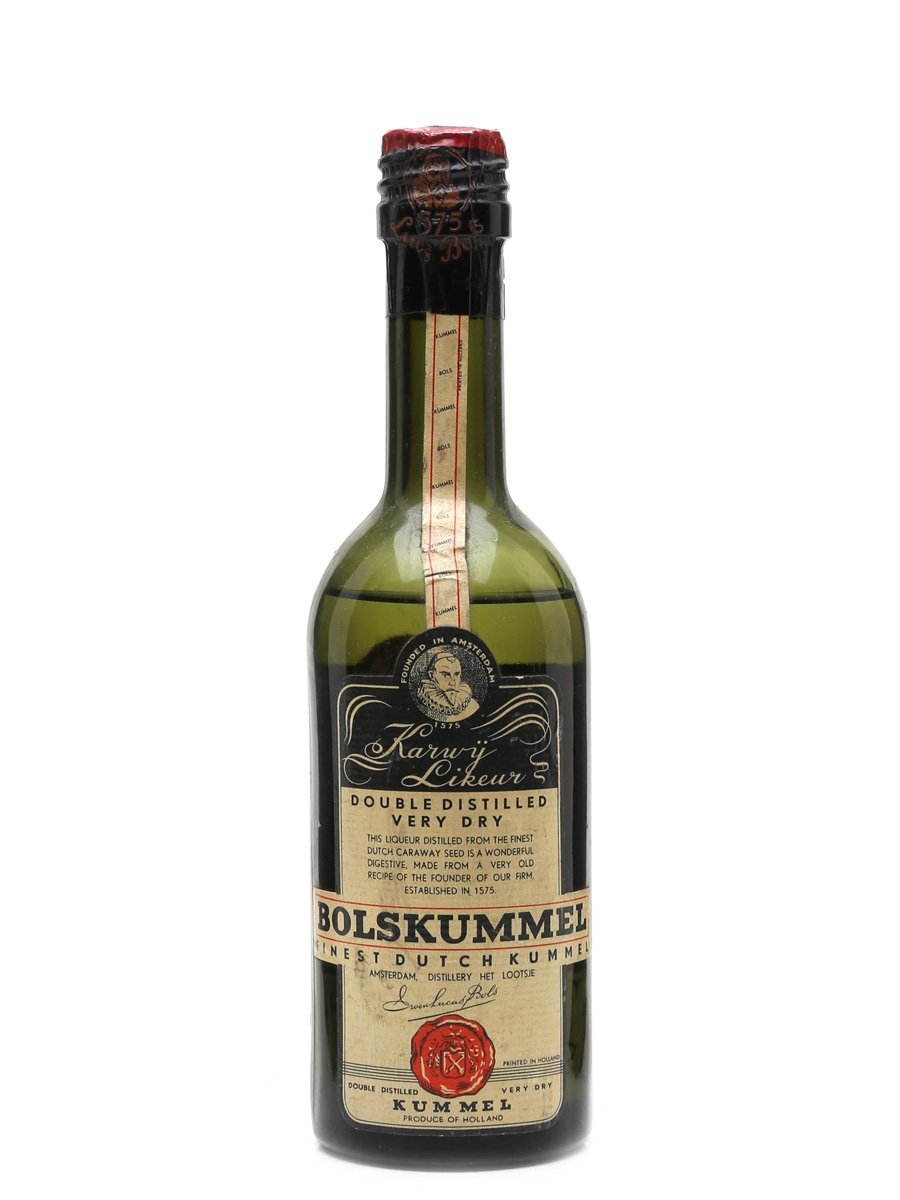This image features a green, unopened bottle of alcohol with intricate details. The bottle is sealed with black tape and capped with red. Just above the cap is a barely visible orange seal featuring a portrait of an old man. Down the neck, a strip of tape with a red vertical line can be seen. The main label, which is black and tan, presents a portrait of a man with a pointy beard at the top in a white cursive script that reads "Carvey Liquor." Below this, in black text, it states: "Double Distilled Very Dry."

The label elaborates: "This liquor, distilled from the finest Dutch caraway seed, is a wonderful digestive made from a very old recipe of the founder of our firm, established in 1575." Dominating the center of the bottle, bold black text on a white rectangle proclaims "Bolskamel, Finest Dutch Kamel, Amsterdam Distillery Het Lutzi." Near the bottle's base, a red wax seal design is followed by the text: "Double Distilled Very Dry, Kamel, Produce of Holland." The bottle is filled approximately three-fifths with liquid, and the background is neutral, devoid of any additional elements.